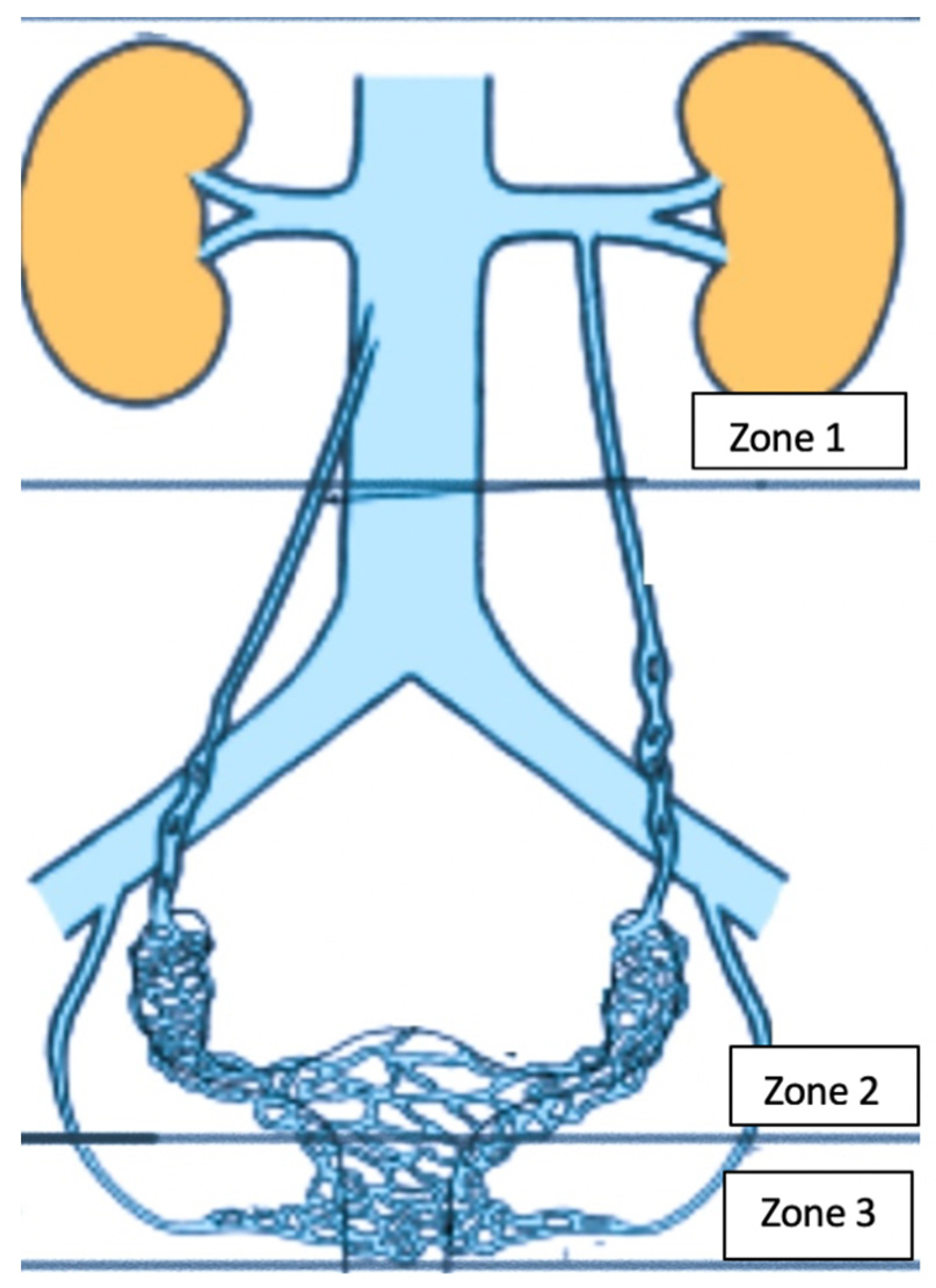The image is a detailed diagram of the internal organs of a human female, primarily focusing on the kidneys and possibly the reproductive and excretory systems. The diagram is divided into three distinct zones. Zone 1, at the top, features a prominent blue vessel, presumably the aorta, which branches out to connect to two orange kidney-like structures on the left and right. These kidneys have blue veins running to them. Alongside these vessels are two cords or ducts that descend from Zone 1 all the way down to Zone 3.

Zone 2, the largest section in the middle, shows the blue tube (aorta) branching off further and also becoming more complex with additional smaller tubes and ducts weaving around. One branch appears to fork over to the left and right. This intricate network likely represents parts of the reproductive system such as the fallopian tubes and uterus, as well as additional vasculature.

Zone 3, at the bottom, is a thin bar that contains the continuation of this intricately woven network of ducts and vessels, corresponding to the pelvic area in the human body. Notably, there are three black lines marking the boundaries of each zone (Zone 1 at the top, Zone 2 in the middle across the uterus, and Zone 3 at the lower region where the opening of the reproductive system is depicted). The color scheme of the diagram includes blue for the primary vessel and veins, dark yellow for the kidneys, and black for the zone demarcations.